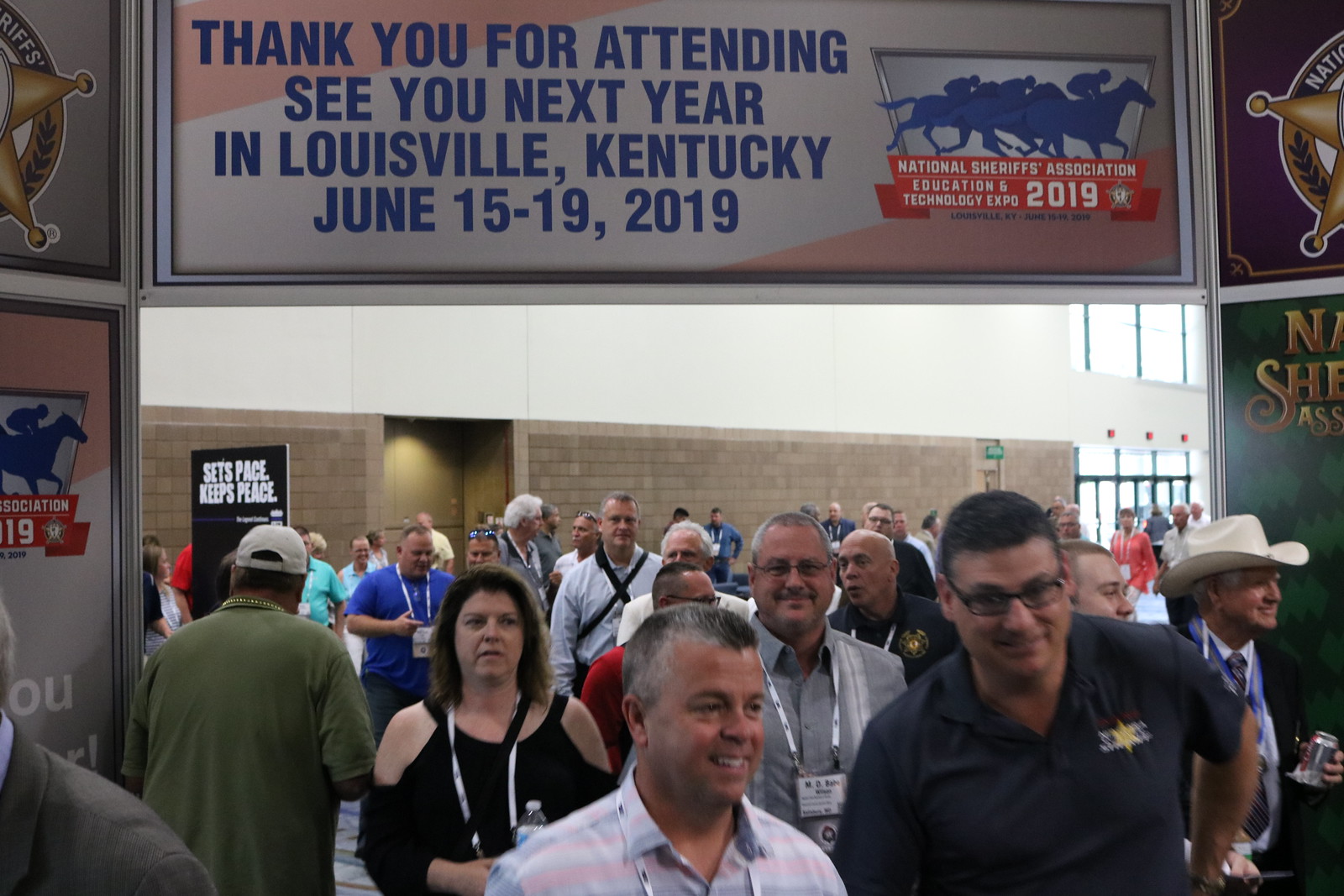The image captures a bustling crowd of people inside a building, seemingly transitioning between areas or exiting. Occupying the foreground are men and women of various ages, all donning lanyards with badges around their necks—one notable man on the right is distinguished by his cowboy hat. The backdrop features a brown brick wall with an overhead sign that reads, "Thank you for attending. See you next year in Louisville, Kentucky, June 15th to 19th, 2019" in blue lettering. Adjacent to this, another banner in a red strip with white text announces, "National Sheriffs Association Education and Technology Expo 2019," accompanied by an abstract blue image of a horse race. A doorway in the brick wall opens into a brighter space where sunlight floods through glass doors and windows, indicating it is daytime. The crowd mingles under the archway, framed by the different textures and tones of the walls, creating a lively and inviting atmosphere as they conclude their visit.